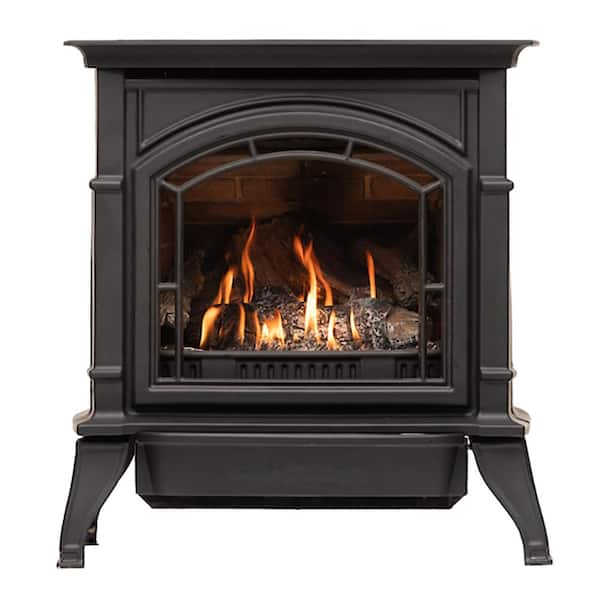This image features a standalone black fireplace made of wrought iron or cast iron, set against an entirely white background, possibly edited for advertising purposes. The fireplace has four legs and a flat top, with a decorative filigree molding around its framed glass door, which appears to be non-functional. Inside, simulated logs sit on a grid with flames of red, orange, and yellow rising from them, suggesting a gas-powered fire. The back of the fireplace includes a brick-like design, enhancing the illusion of a traditional wood-burning hearth, while the glowing embers illuminate the surroundings, indicating the logs are charred. A tray beneath the fireplace likely facilitates adding kindling or lighter fluid.